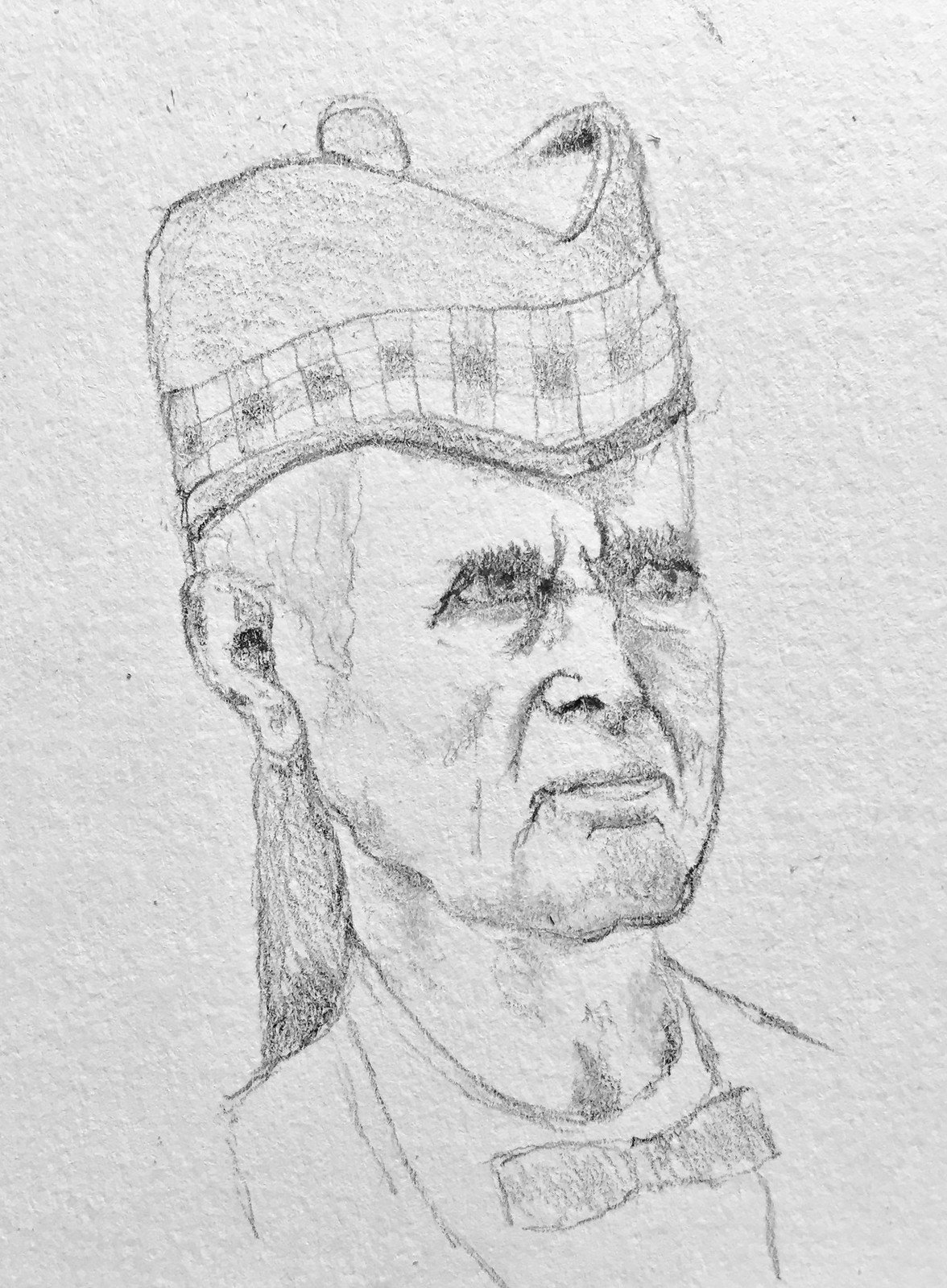The image depicts a highly detailed black and white sketch on textured, wrinkled paper. The subject is a man whose upper torso and face are prominently featured. He is wearing a unique, pointed cap with a checkered trim and shaded black edging. This hat, which has a V-cut in the front, extends down near his nose and rises back up. The man has a pensive expression, characterized by his furrowed brows and bushy eyebrows, giving him an older, somewhat angry appearance. His face is well-defined with wrinkles around the mouth and cheeks, and he sports what appears to be a small beard on his chin. His hair is pulled back, possibly into a ponytail, revealing a balding top. The man's attire includes a bow tie paired with what seems to be a high-collared shirt or t-shirt and a jacket. Despite the minimalist color scheme, the shading and texture of the drawing, enhanced by the textured surface it's on, bring a vivid depth to the sketch.